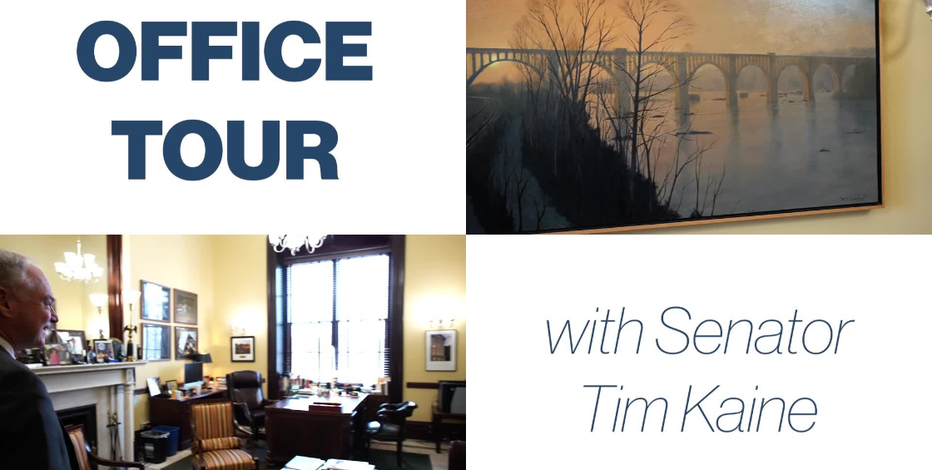The image is a probable PowerPoint slide set in a landscape orientation, divided into four equal rectangles - two on the top row and two on the bottom. The top left rectangle features a white background with blue text that reads "Office Tour." To its right, the top right rectangle contains a photograph of a framed picture depicting a bridge, surrounded by water, trees, and bushes, set against a cream-colored wall. Below, the bottom left rectangle showcases an image of an office with cream-colored walls, a desk with a chair, and a white fireplace. In this office, an older, balding gentleman stands smiling, facing the interior with a window in the background. The bottom right rectangle, also with a white background, displays light blue text that reads "With Senator Tim Kaine (T-I-M K-A-I-N-E)."